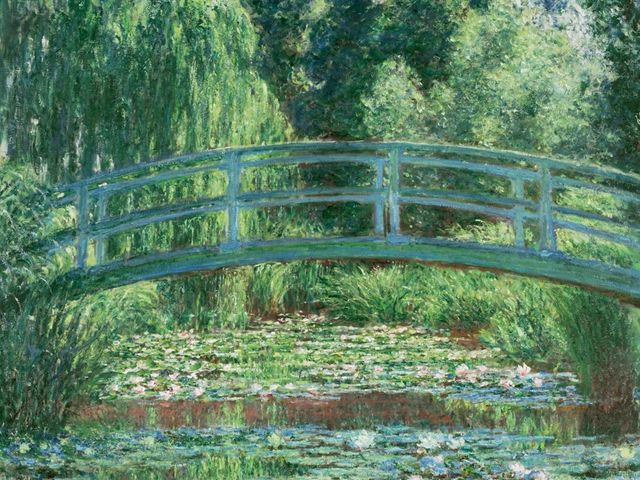This detailed oil painting meticulously captures an idyllic, secluded scene, showcasing a small, naturally arched wooden walking bridge that spans across a lily pad-filled pond. The bridge, primarily blue and green with touches of white, seamlessly blends with the surrounding flora, suggesting it's been overtaken by nature. Above and behind the bridge is a dense, thickly forested area with a variety of green shades mixed with yellows and slightly darker hues. The top of the image is dominated by tall trees and lush vegetation, creating a natural canopy that filters light into the scene, giving a natural outdoor ambiance. Beneath the bridge, the water surface is adorned with green lily pads and delicate white and pink flowers. The water itself appears to brim with grass and other aquatic plants, hinting at an overgrown, serene, and untouched environment. The absence of animals, people, or text adds to the tranquility and timelessness of this hidden gem in a wooded park.